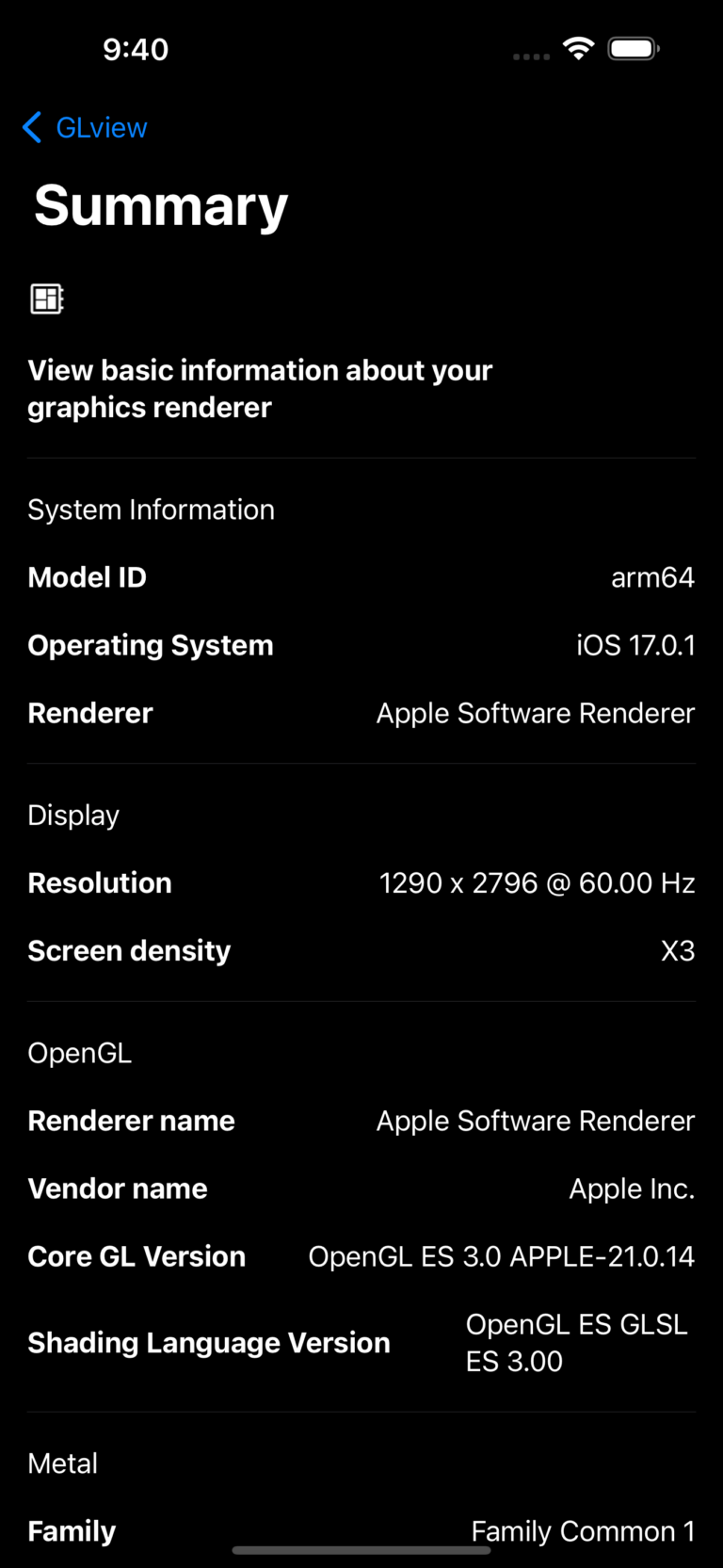The image is a screenshot featuring a minimalist interface with a black background and white text. In the top-left corner, the word "GLView" is displayed in blue text, accompanied by a blue back arrow. Below this, the word "Summary" appears in large, bold, white lettering. The remaining information is presented in smaller, uniform white text. 

The screen details various technical specifications, as follows: 
- A heading under "Summary" indicates "view basic information about your graphics renderer."
- System Information lists:
  - Model ID: ARM64
  - Operating System: iOS 17.0.1
  - Renderer: Apple software renderer
  - Display Resolution: 1290 by 2796 at 60.00 Hz
  - Screen Density: X3
  - OpenGL Renderer Name: Apple software renderer
  - Vendor Name: Apple Inc.
  - Core GL Version: OpenGL ES 3.0 Apple-21.0.14
  - Shading Language Version: OpenGL ES GLSL ES 3.00
  - Metal Family: Family Common 1

All details are set against a simple black background, utilizing clean, white text for clarity.